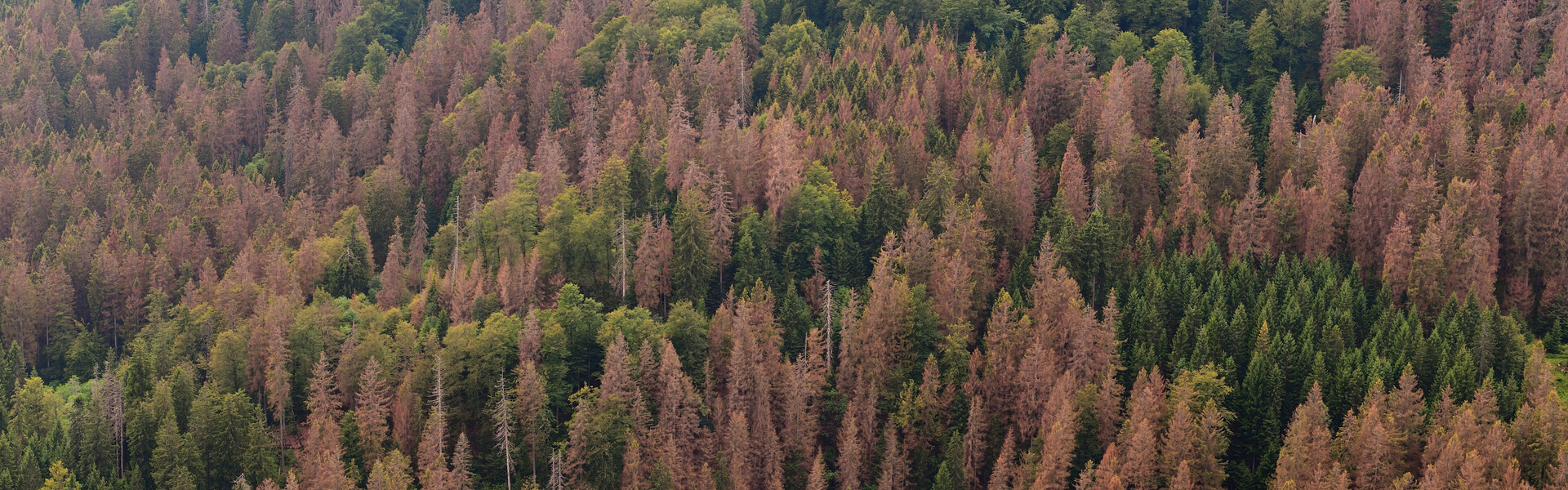This image captures a wide, horizontally-oriented landscape of a dense forest on an autumn day. The photo, seemingly taken from above by a drone or aircraft, offers an aerial perspective that reveals only the tops of numerous trees. These trees are a mix of green and brown, with the green trees showing dark, shadowy areas beneath their canopies and the brown trees appearing somewhat dead, lacking leaves and exposing their branches. The forest appears continuous and vast, almost blending into a distant spiked terrain-like pattern in the upper center of the image, where smaller trees are interspersed among the taller ones. The scene's composition, focused exclusively on the tree canopies, omits the forest floor, emphasizing the tops' dense, uniform spread and the contrasting colors.